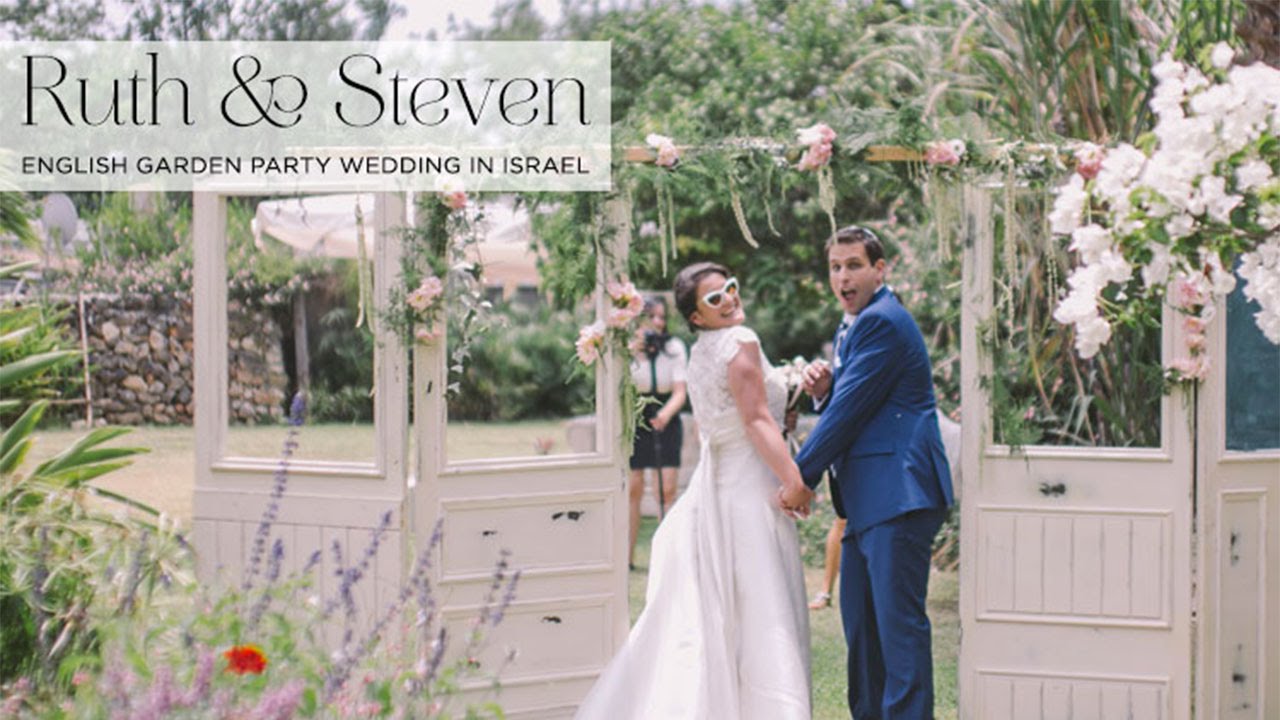In the image, a couple who appear to have just been married are standing in front of a vintage photography backdrop composed of connected, cream-colored doors, adorned with pink and white flowers framing the top. The bride is dressed in a white wedding gown and is wearing white sunglasses, while the groom is in a navy blue suit and sporting a Jewish head covering. They are holding hands and looking back towards the female photographer, who is dressed in a white short sleeve top and a black skirt. The backdrop is set in a lush garden filled with greenery, including trees, shrubs, and plants in various colors like green, blue, and purple. In the background, there is a small stone wall to the left. On the top left corner of the image, text reads "Ruth and Stephen, English Garden Party Wedding in Israel" in black font on a slightly transparent white background, indicating it may be used for invitations or a wedding website banner. The overall scene exudes a vibrant and joyous wedding atmosphere.